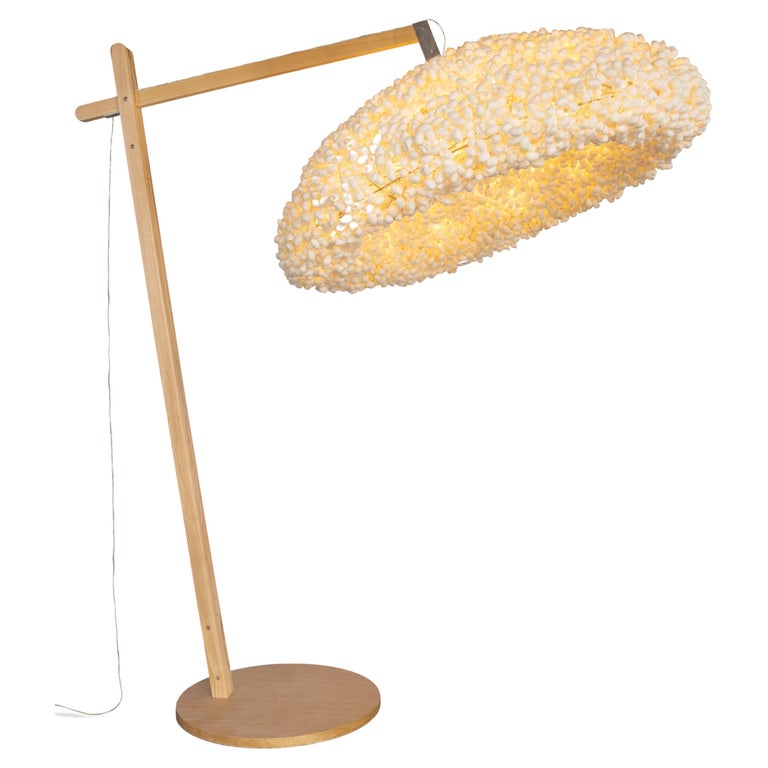This image shows a stylish floor lamp set against a white background. The lamp features a round, flat wooden base made of light-colored, unfinished wood. A thin, slightly tilted wooden pole extends upwards from the base, connected to a horizontally inclined wooden arm. This arm is secured to the upright pole with visible small nails. At the end of the horizontal arm, a short metal piece angles downwards, supporting a unique lamp shade. The shade appears to be covered with a textured, furry-like material, potentially resembling cotton or small pieces of styrofoam balls, all in a cream color. The lamp is lit, casting a warm yellow glow that accentuates the texture of the shade. Additionally, a black cord is visible near the connection point of the wooden components, trailing down to the surface below.